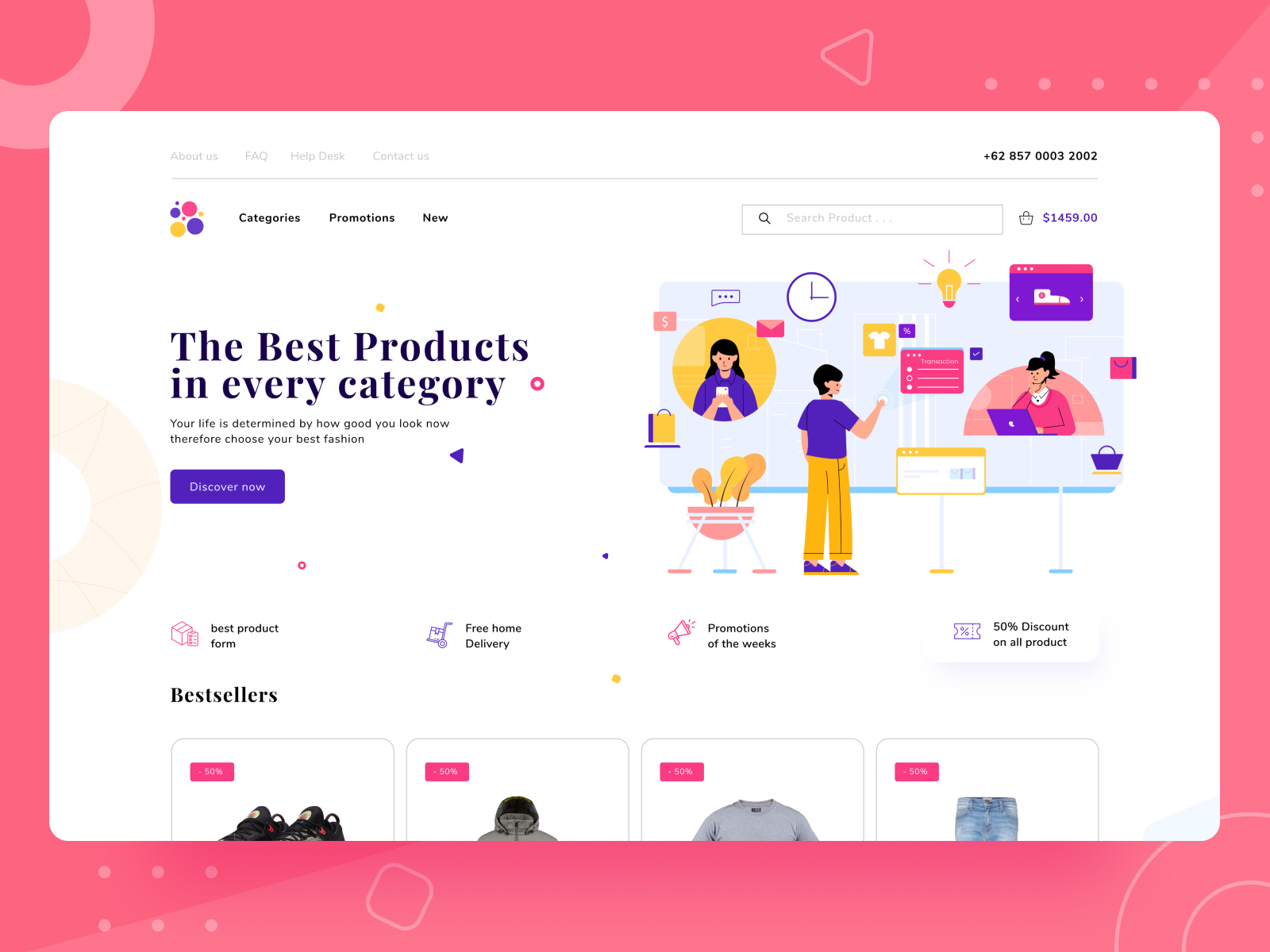The image features a vibrant and busy scene filled with various elements. Against a pink background adorned with lighter pink circles, a small triangle, and several dots, the central focus is a white inset near the top displaying the number "+62857000032002". 

On the left edge, four large balloons in blue, pink, and yellow are accompanied by three smaller balloons. Below this, there's a search box with a magnifying glass, and beside it, a purple text proclamation states, "The best products in every category." Nearby, a pink circle highlights the inspiring message, "Your life is determined by how good you look now therefore choose your best fashion."

A prominent blue button labeled "Discover Now" features a left-facing arrow. Adjacent to this is a small section promoting "Best Product Form," illustrated with a box drawing, "Free Home Delivery," and a "Promotions of the Week" banner announcing a "Fifty Percent Discount on All Products."

To the right, at the top, a price tag displays "$1,459" in purple. Below, there's an image of a girl wearing purple inside a yellow box, holding a white paper. Above her, a pink box features a dollar sign. Nearby, an envelope, a purple and yellow shopping bag, and a pink planter with three yellow plants add to the scene.

Further right, a lady dressed in yellow pants and a purple top stands near a clock showing three o'clock. There's a yellow square displaying a white shirt, a pink sign, a light bulb, and a purple sign topped with pink. Seated at a desk with a purple computer, another lady in pink completes the office scene.

At the bottom, under the "Best Sellers" section, four products are showcased, each marked by pink boxes indicating their prices.